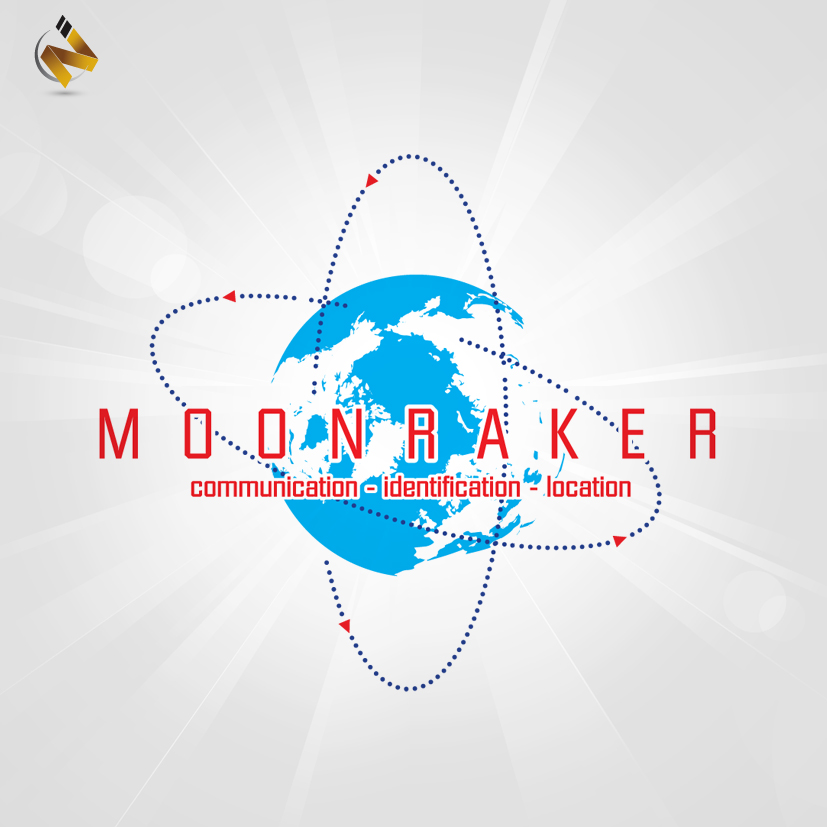This image features a flyer predominantly set against a gray background, with dynamic design elements drawing the viewer's attention toward the center. The focal point consists of text that reads "Moon Rica Communication Identification Location," situated centrally over an emblematic depiction of the Earth. The globe is illustrated in blue and white, emphasizing land and sea, and is encased by elliptical lines indicating latitude and longitude, also rendered in blue. These ellipses are accentuated by blue dots, adding a sense of depth and movement.

Radiating from the center of the image are white rays, creating an eye-catching effect that directs attention toward the central text and globe. Positioned in the top-left corner is a distinctive logo, characterized by an inverted letter "N" in a vibrant yellow hue.